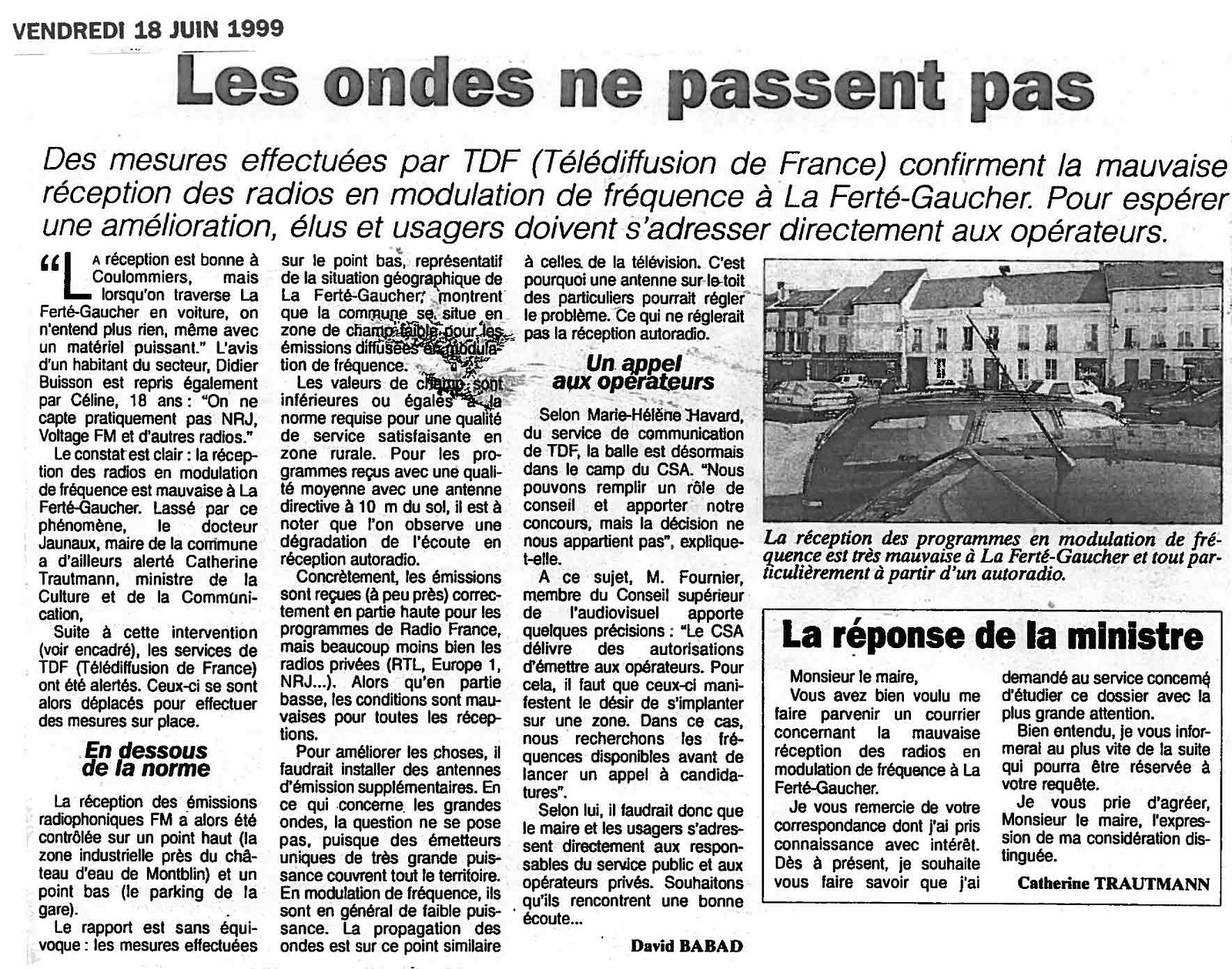This image captures a photocopied page of a French newspaper from June 18, 1999. The white background clearly frames a meticulously laid-out article, which is composed of about five or six paragraphs and formatted into two distinct sections. Prominently titled in bold black text, the piece also features a boxed subsection located beneath a black and white photograph on the left side. This photograph appears to depict a group of buildings, possibly townhouses, with around nine cars of varying positions parked in front of them. The top left corner distinctly displays the date, "Vendredi 18 Juin 1999," establishing the timeframe of the publication. Despite some smudging of the text, certain words like "réception," "programmé," and "modulation" are visible, along with the names Catherine Troutman and David Babad. The overall appearance suggests the article discusses a local event or program, possibly related to a venue where cars are prominently involved.